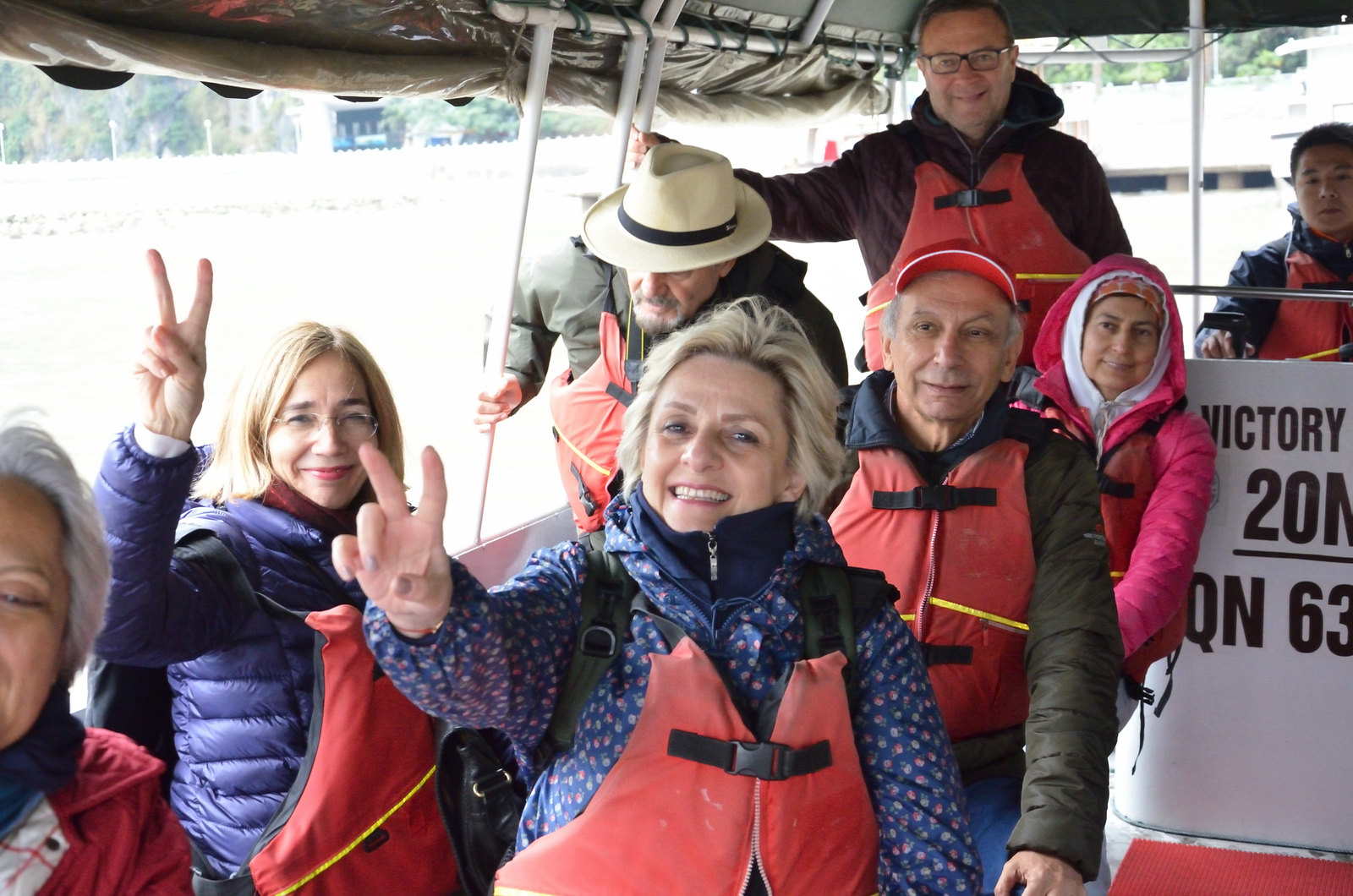The photograph captures an outdoor scene on a boat with a group of eight people, all bundled up in winter jackets and red life jackets that appear worn. In the foreground, two blonde women, likely white, pose with cheerful peace signs directed at the camera. Behind them, two men in hats and life jackets stand, with one of the men flanked by a woman in a pink coat and hoodie, also donning a life jacket. A tall white man with glasses and a dark-colored hoodie stands nearby, alongside an Asian man in a black jacket. The boat exterior is a blinding white, reflecting sunlight and the surrounding water’s glare, with a glimpse of greenery visible in the distance. On the right-hand side, partially cropped but readable in brown font, is a sign with the text "Victory 20 QN63". It seems the group is ready to embark on a voyage.